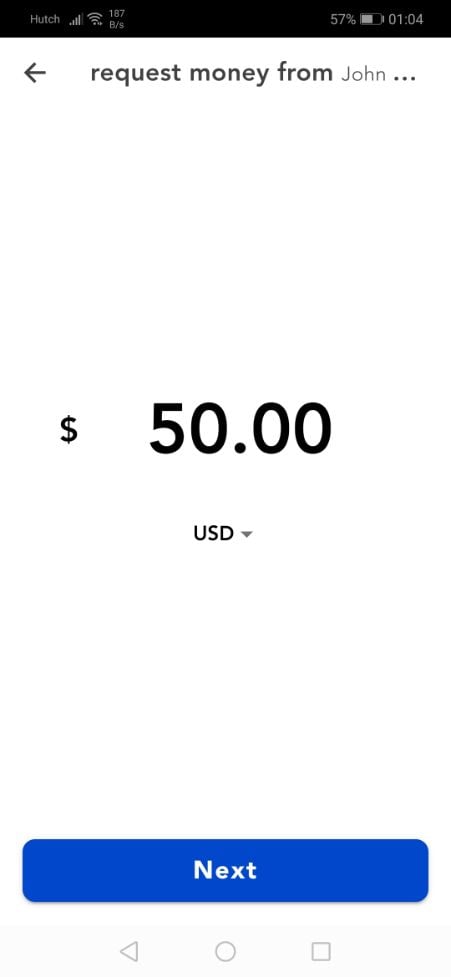This detailed caption describes a screenshot of a payment application displayed on a smartphone screen in portrait orientation.

---

**Caption:**
The screenshot showcases a payment app interface on a smartphone. The image has no defined borders and presents a complete view of the app's screen.

**Top Bar Details:**
- A horizontal black bar spans the top, containing several status indicators in grayish text:
  - "Hutch" is displayed on the left, possibly indicating the app's brand.
  - An internet connection meter shows full signal strength.
  - A Wi-Fi meter also indicates full connectivity.
  - "187 bits per second" appears to denote the current data transfer rate.
  - On the right side, a "57%" indicator shows the remaining battery life, accompanied by a battery icon.
  - The time displayed is "01:04."

**Header Section:**
- Below the status bar, a header includes:
  - A back arrow on the left.
  - The text "Request money from" in black, followed by the name "John" in gray.

**Main Content:**
- In the center of the screen, a dollar sign and the amount "$50" are visibly displayed.
  - The currency is set to "US dollars," with a dropdown menu available for selecting other currencies.

**Navigation and Action Buttons:**
- Below this, a blue rectangular button with rounded edges is labeled "Next" in white font.
- At the bottom, there is a navigational bar featuring three icons: a back arrow, a circle, and a rectangle, suggesting typical smartphone navigation options.

The app appears designed for requesting monetary transactions.